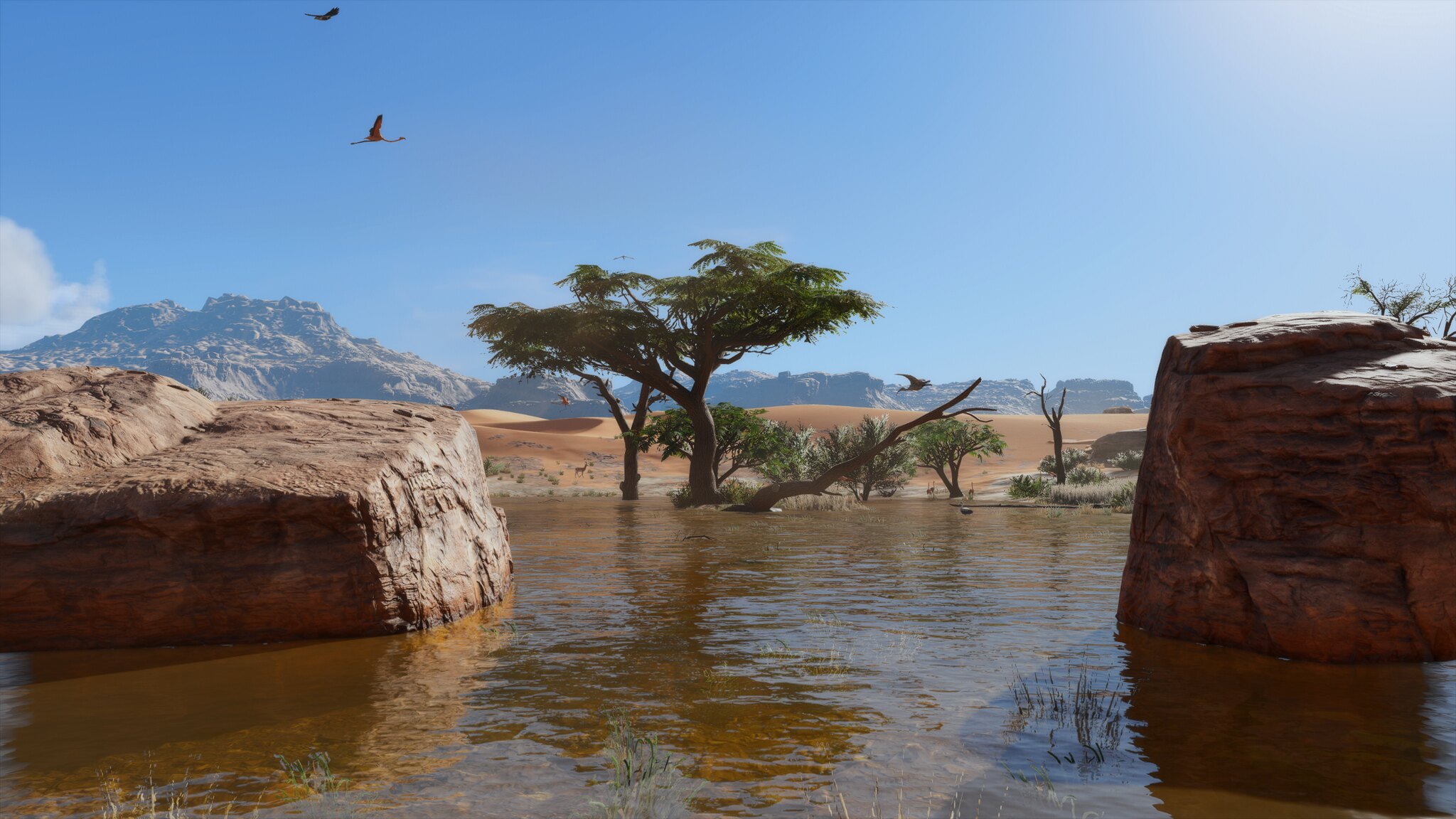This is an animated, AI-generated image of a picturesque outdoor landscape. Dominating the scene are two towering boulders on either side, partially submerged in a reflective, brownish body of water. Towards the center, a large, lush tree with a flat, expansive canopy rises from the water, its foliage casting a greenish-brown tint. The water is shallow and dotted with patches of grass.

In the background, a series of undulating sand dunes stretch across the desert-like terrain, leading to a range of rocky, sparsely vegetated mountains. These mountains display layers of dark and brown highlights, giving them a rugged, textured appearance.

Above, a brilliantly blue sky extends across the scene, with the sun casting its bright rays from the upper right corner. A single wispy white cloud drifts on the left, adding a touch of softness to the otherwise clear expanse. Soaring through the sky are several bird-like creatures resembling dinosaurs, with long, thin necks and expansive wings, while one bird stands out with its pink hue and elongated legs trailing behind it.

This captivating landscape, with its blend of natural elements and vivid details, exudes the essence of a serene savannah desert.